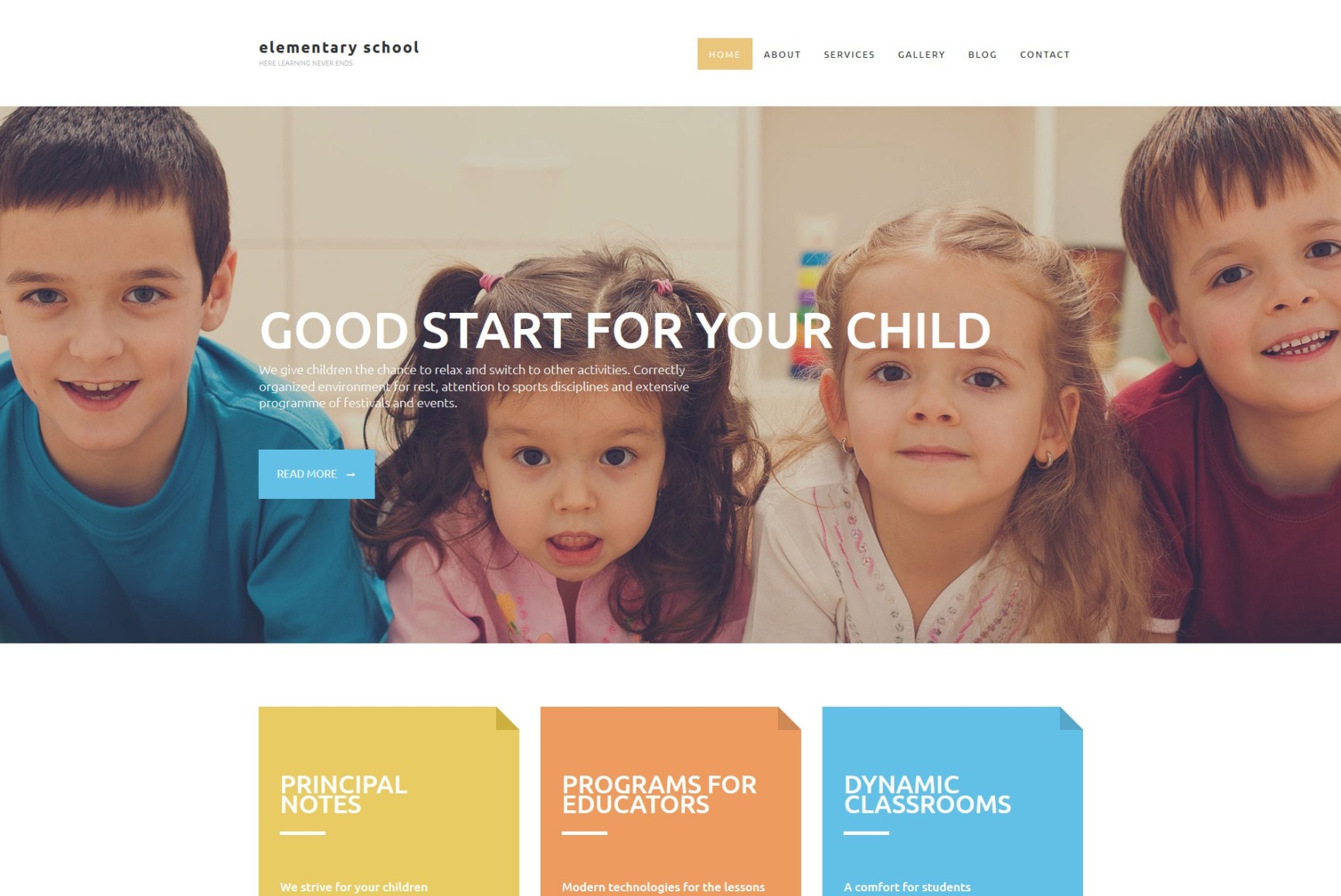**Website Banner Description: Detailed Elementary School Landing Page**

At the top of the webpage banner, black lowercase letters spell "Elementary School." Below this heading is a smaller line of black text that is too tiny to be legible. On the right-hand side, a tan rectangle contains the word "Home" in white lettering. Adjacent to this, a row of black labels lists "About," "Services," "Gallery," "Blog," and "Contact."

Beneath this navigation bar, a full-width rectangular image spans from edge to edge. Across its center, bold white lettering proclaims the message "Good Start for Your Child." The image features four young preschool-age children: a boy on the left, two girls in the center, and a boy on the right. 

To the left side of the text, a blue rectangular button with white lettering encourages viewers to "Read More." Below the main text, a small paragraph of white text provides additional context or information.

At the bottom of the banner, three square icons resemble tipped landscape sheets of paper with dog-eared upper right-hand corners. The first icon is tan or yellow with bold white text stating "Principal Notes." The second icon is light orange with white text that reads "Programs for Educators." The third and final icon is turquoise blue, featuring white text that says "Dynamic Classroom."